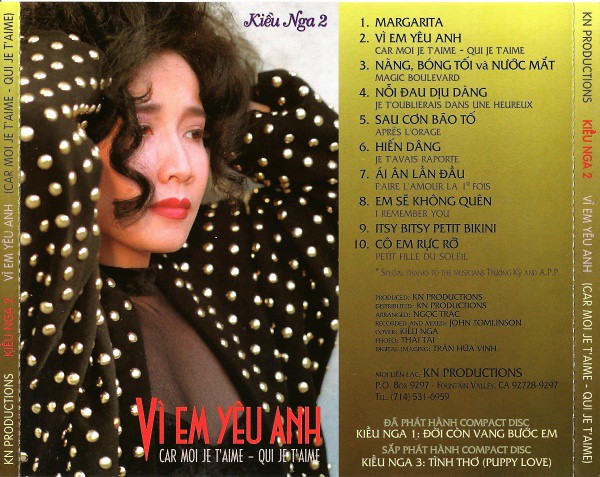The album cover features a striking image on the left side, dominated by a photograph of an Asian woman with curled hair, looking to the right with a notably upset or sad expression. Her attire is distinctive: she wears a black coat embellished with numerous silver metal studs, layered over a semi-sheer black shirt and a solid black collar. She has black lipstick, which further emphasizes her dramatic look. The right side of the cover features a gradient gold rectangle, transitioning from a darker gold at the bottom to a lighter yellowish gold at the top. There is also a shorter gradient gold border on the far left side. At the top middle of the album, text reads 'K-I-E-U-N-G-A-2.' Below her image, text displays "V-I-E-M-Y-E-U-A-N-H" and "C-A-R-M-O-I-J-E-T'J-A-I-M-E-Q-U-I-J-E-T-A-I-M-E." The right side includes a listing of ten tracks, starting with "Margarita" at the first position and ending with "Puppy Love" at the very bottom. The production credits and album details are noted below the track list. The cover is attributed to KN Productions.